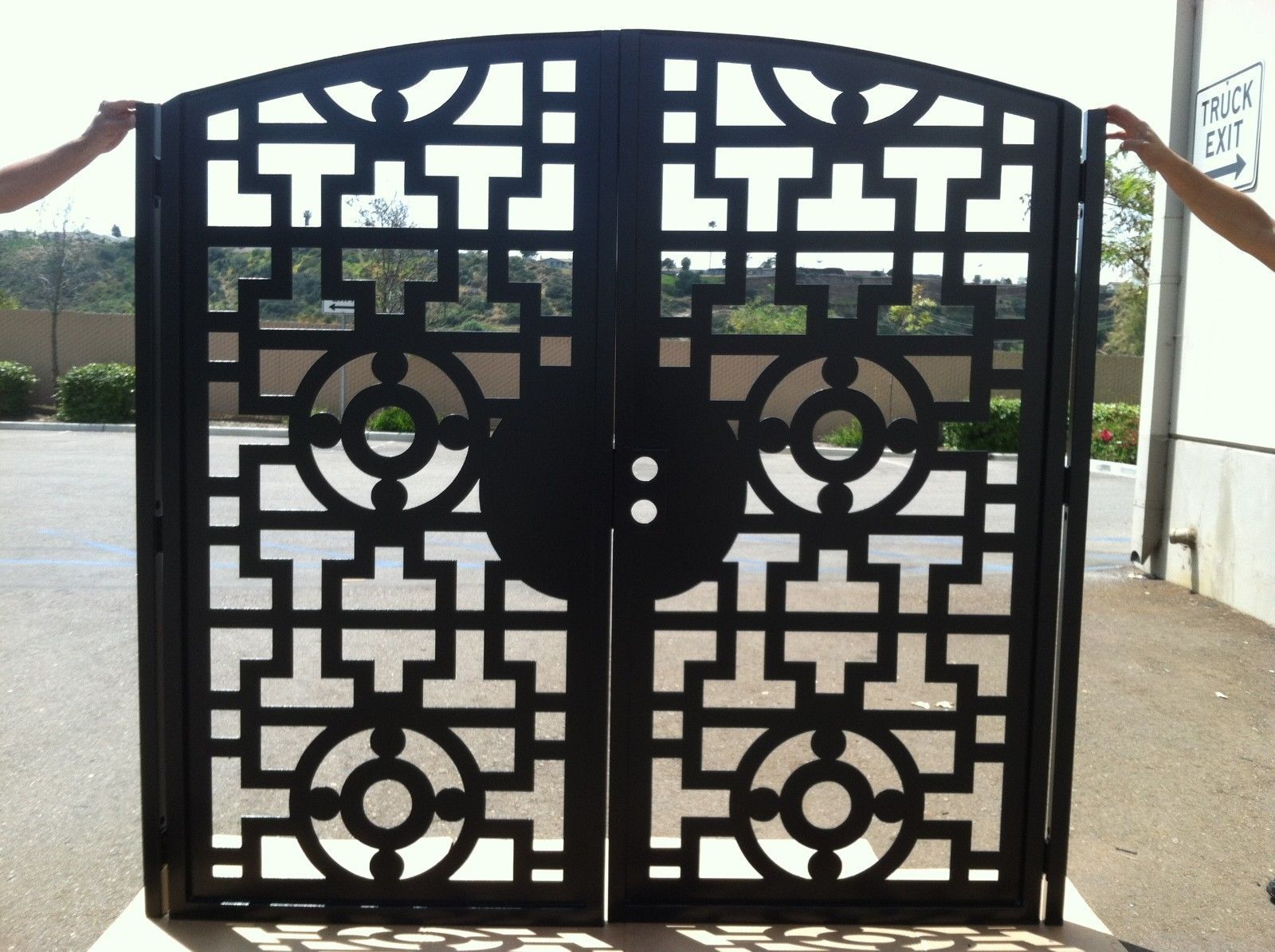In this detailed image, we see two human hands holding up an uninstalled black metal gate designed for an entrance doorway, positioned outdoors. The gate is divided into left and right sections and features decorative lattice work with circular patterns and lines, making it see-through in the middle areas. The top of the gate is curved while its sides and bottom are flat. The scene appears to be taking place in a back alley or behind a warehouse, evidenced by the gray cement floor and white cardboard sheet underneath the gate. On the right side, a white building bears a sign reading "truck exit," pointing to the right. In the background, there is a brown fence, some trees, and a white, overcast sky. The hands are positioned at the top left and top right corners of the gate, indicating that it is likely being reviewed or shown for demonstration purposes.